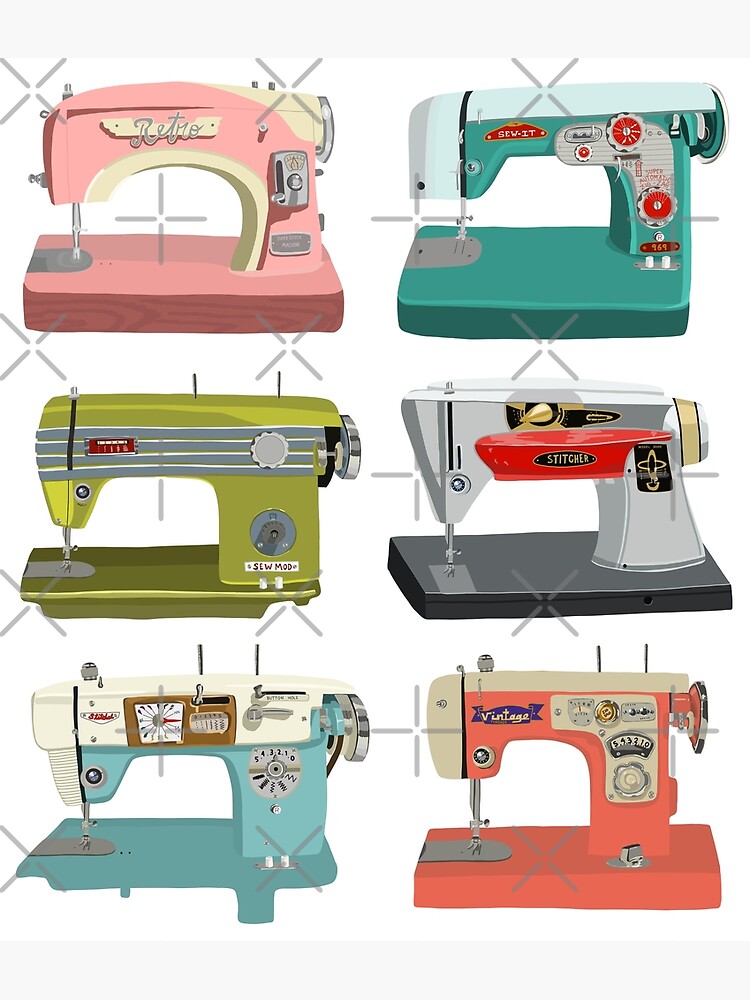The image is a detailed, colorful clip-art illustration of six fanciful sewing machines against a white background. These machines are arranged in two columns, each with three sewing machines, making a total of six. The illustration features dashed X's, signifying it may be a preview of a transparent background clip-art.

Starting from the top left, the first sewing machine is pink with cream-colored accents and a tan trim, labeled "Retro," with a coin slot-like feature. To its right is a turquoise machine with aqua accents and a metal manufacturer's plaque featuring red stripes and circular appliques. 

In the middle row, the left machine is avocado green with a gray or silver broad stripe and a riveted red manufacturer's label. Adjacent to it is a futuristic-looking silver machine with red, black, and gold accents, and a distinct black base.

The bottom row hosts a light blue machine with a white top and a square clock or radio-like feature, though the brand is indiscernible. Lastly, on the bottom right, there is a coral pink sewing machine with a cream top, adorned with a blue ribbon-shaped tag that reads "Vintage."

The image stands out with its vivid colors and realistic shading, lending visual interest and a touch of nostalgia with its retro-themed designs.